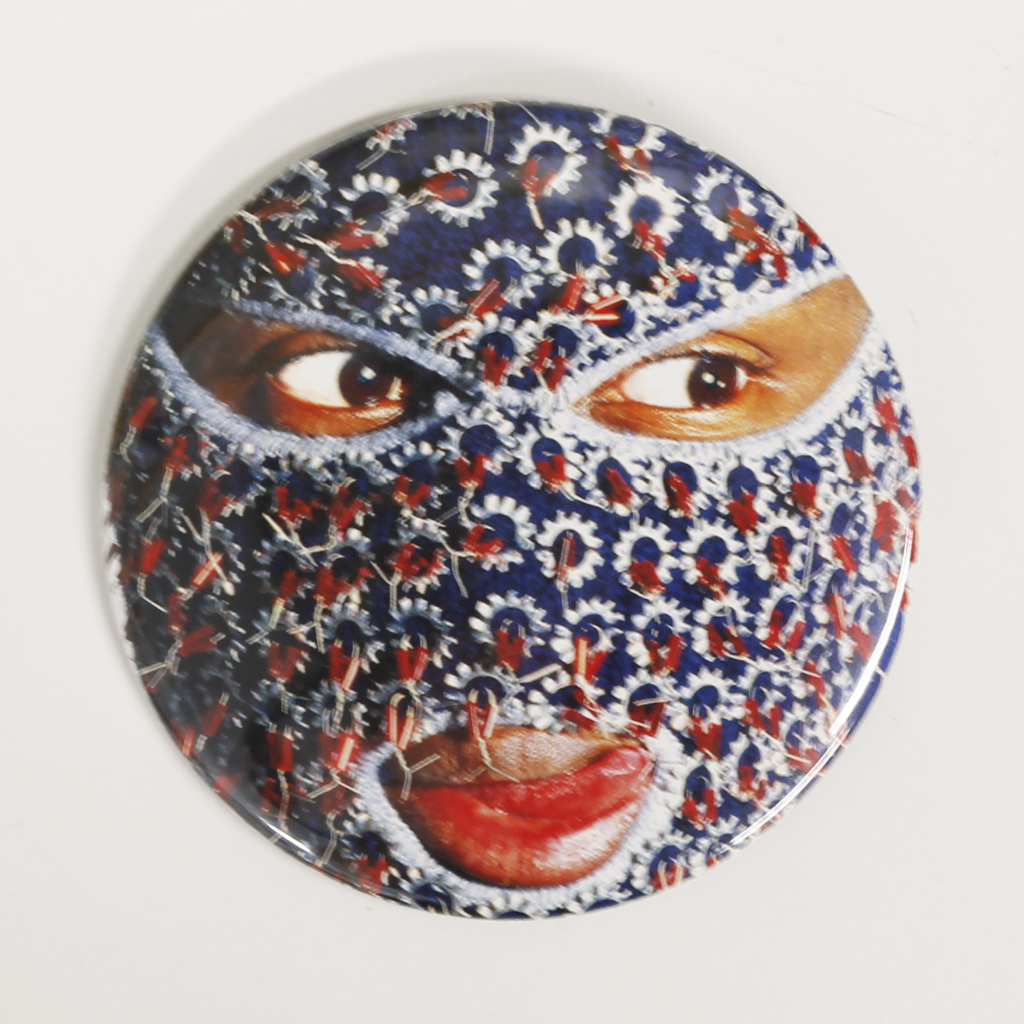The image is a color photograph of a circular pin with a glossy finish, featuring a human face mostly covered by a navy blue ski mask adorned with a repeating pattern of white gear-like shapes, each with red strings or stylistic designs at their centers. The background of the image is a light gray or off-white, and the circle nearly fills this square background. The mask has cutouts for the eyes and mouth, revealing brown eyes that gaze to the right and broad lips with a tongue protruding slightly to the right. The eyes, mouth, and tongue add an expressive element to the image, which combines red, white, and blue colors prominently on the mask, creating a striking visual contrast against the light base.